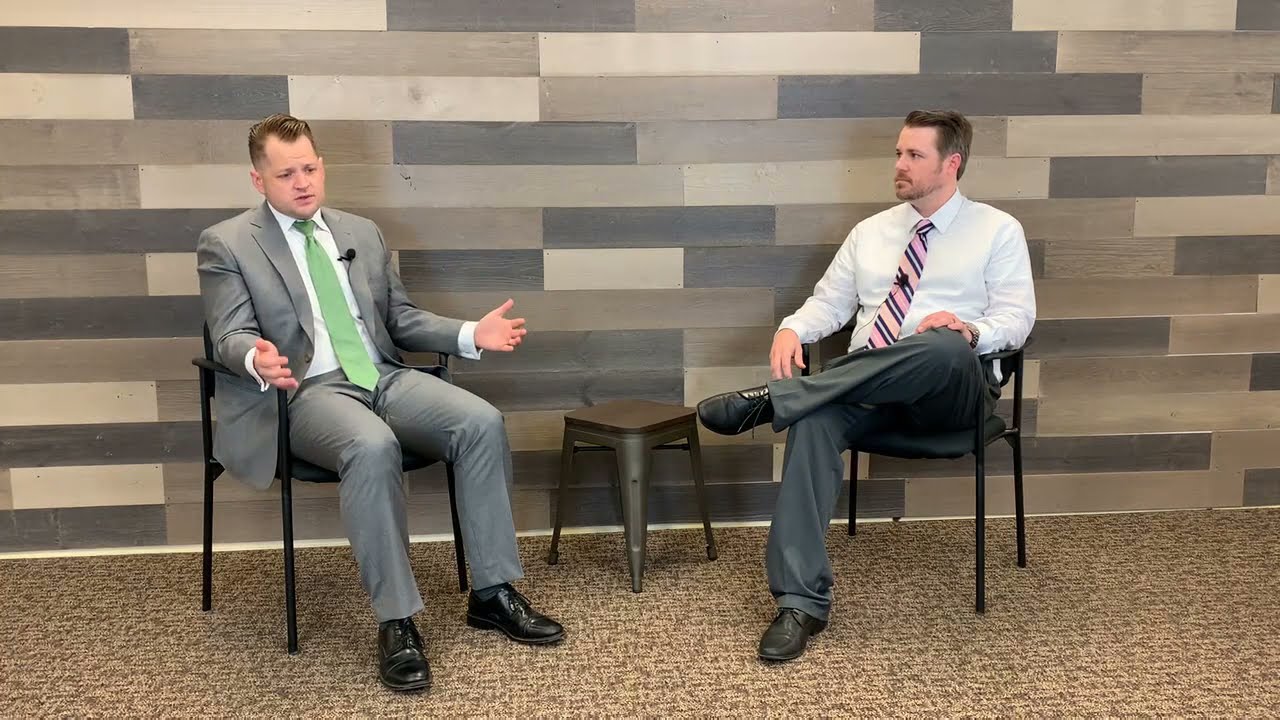In this business-related image, two middle-aged men are engaged in a conversation, likely part of an interview or podcast, seated in black chairs in front of a backdrop made of multicolored rectangular wood panels in shades of blue, grey, and tan. The floor beneath them is carpeted in varying shades of brown, differentiated from the wall by a white baseboard. The man on the left, who has short brown hair and a clean-shaven face, is dressed in a gray suit with a mint green tie, gray pants, and shiny black leather shoes. He appears to be gesticulating as he speaks, with his hands open, palms up. The man on the right, also with short brown hair but sporting a goatee, is wearing a long-sleeved white button-up shirt paired with a pink and black diagonal-striped tie, dark gray pants, and black leather shoes. His left leg is crossed over his right, and he is engaged in the discussion, looking towards his companion. The scene is calm and professional, centered around an empty stool positioned between them.